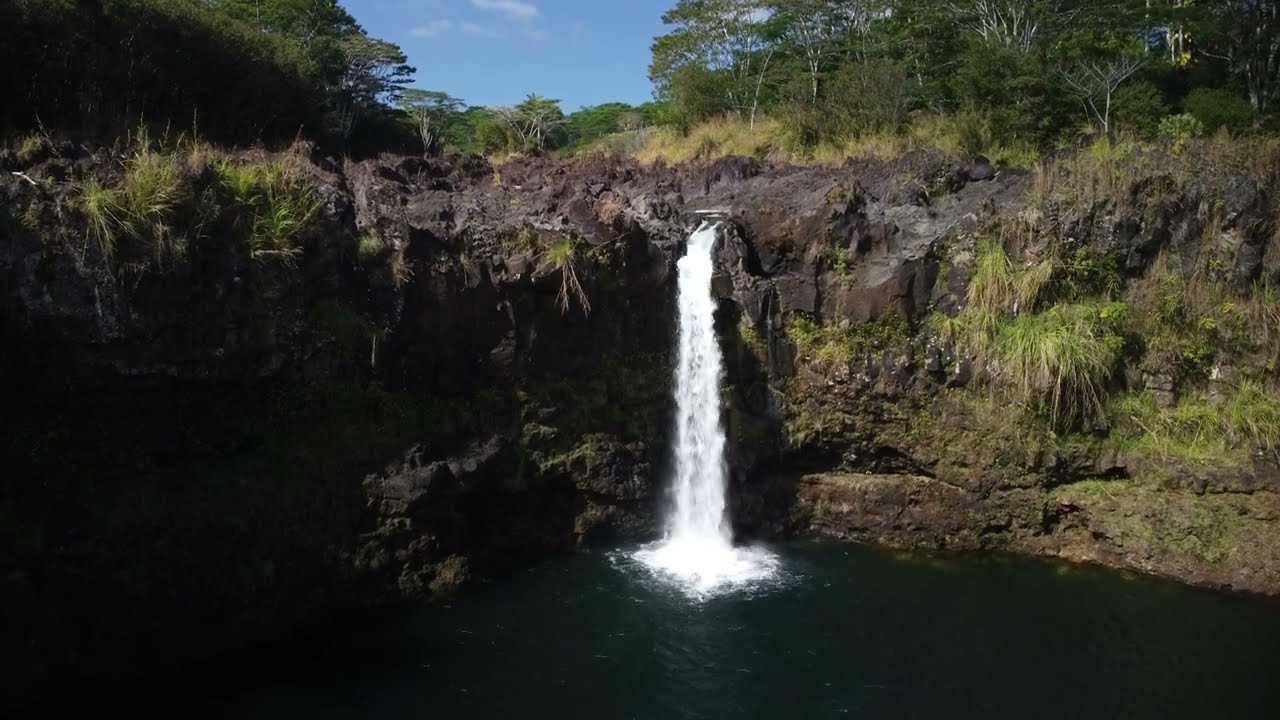The image depicts a stunning medium-sized waterfall cascading down a rocky cliff adorned with lush green vegetation. The waterfall, which stands around 100 to 200 feet tall, is composed of pristine white water that rushes down the side of the cliff, splashing into a dark body of water below, possibly a lagoon or ravine, with semi-transparent edges that reveal some of the underlying rock. The rock face surrounding the waterfall is a dark brown, with hints of reddish and light gray hues, curving around the back of the image and creating a shadowy effect on the left side, while the right side is bathed in sunlight, highlighting the vibrant green grass and bushes. Above the cliffs, the scene transitions into a densely treed landscape, predominantly featuring deciduous trees, set against a light blue sky with a few scattered white clouds. The top of the waterfall is particularly rugged and craggy, contributing to the dramatic and picturesque quality of the scene. No people or animals are visible in the image, focusing attention on the natural beauty and tranquility of the waterfall and its surroundings.